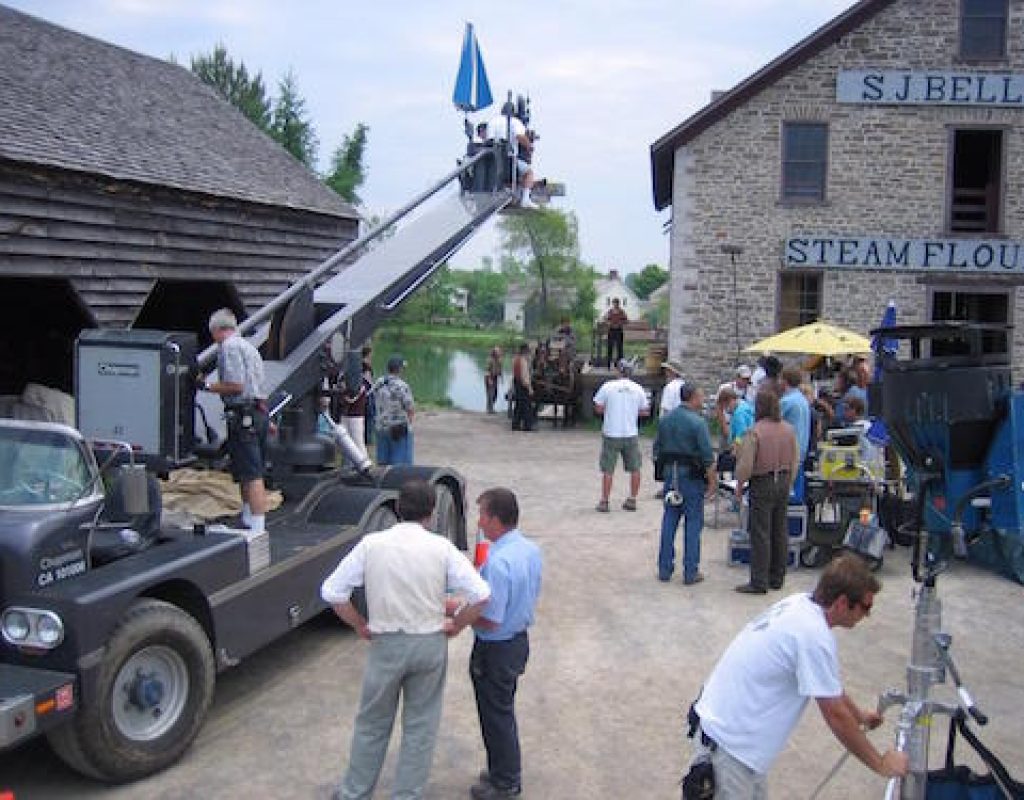This photograph vividly captures a bustling outdoor movie set situated between two old-fashioned, brick buildings. On the left side of the image, a large gray truck with a towering boom lift extends upwards, culminating in a bucket where a man is seated, operating a camera under a closed blue umbrella. To the lower right, another man leans over a hefty tripod topped with what seems to be an industrial light. The right-side building prominently displays the faded sign "S.J. Bell" above partially obscured markings "Steam Flow," hinting at its historical past. In the scene's center and beyond, a serene lake flanked by white houses and deciduous trees lies under a partly cloudy sky. Scattered across the dirt-laden set, crew members in Western attire, including cowboy boots and hats, diligently manage equipment and props like a horse and wagon. A cluster of personnel gathers around a table shaded by a yellow umbrella, reinforcing the collaborative atmosphere of this cinematic endeavor. Colors of green, blue, black, brown, red, and gray contribute to the image's rich visual tapestry, capturing both the filmic process and its rustic setting.